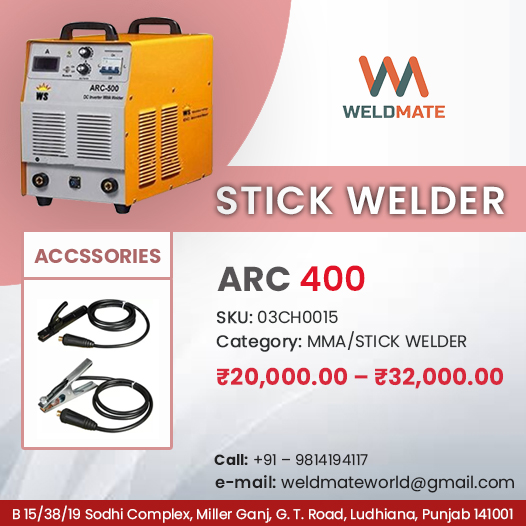The advertisement features a prominently displayed rectangular yellow and white welding machine with several knobs, black handles on top, and vents on the front and side. This machine, labeled as an ARC-500, is central to the ad. To the right, there is a logo for "WELDMATE" in orange and green, with a distinctive combined "W" and "M" design. Below the logo, the machine is described as a "STICK WELDER," with the model "ARC-400" and a SKU number. Additional details include a range of values, "20,000 to 32,000," suggesting specifications or pricing, along with contact information comprising a phone number, email address, and store address. On the left, the ad lists accessories, featuring items resembling clamps or jumper cables. Notably, there is a typographical error in the word "accessories."